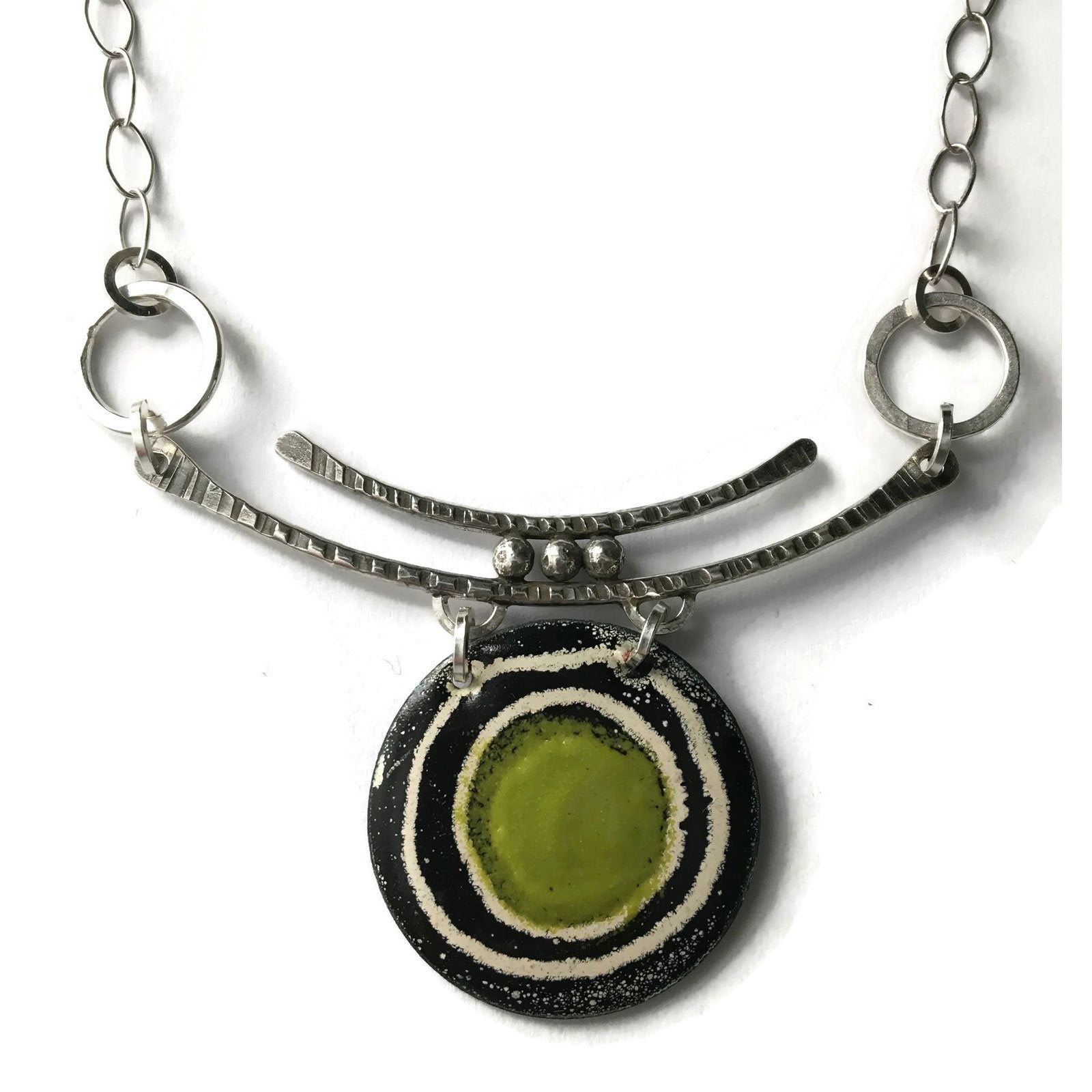The image depicts a distinctive piece of jewelry, set against a solid white or slightly off-white background. At its center, there's a large U-shaped metal bar from which two small silver rings dangle, each attached to a slender silver chain. Above this bar, three metal bearing balls connect to a smaller U-shaped metal piece. Prominently hanging from the larger U-shaped bar is a circular pendant with intricate details: the outer layer is black with a tan ring enclosing another tan circle, which itself encircles a green glass-like interior. The overall design evokes an artistic, possibly cultural aesthetic, reminiscent of Native American or Greek jewelry, featuring a combination of delicate chains and striking pendant elements.